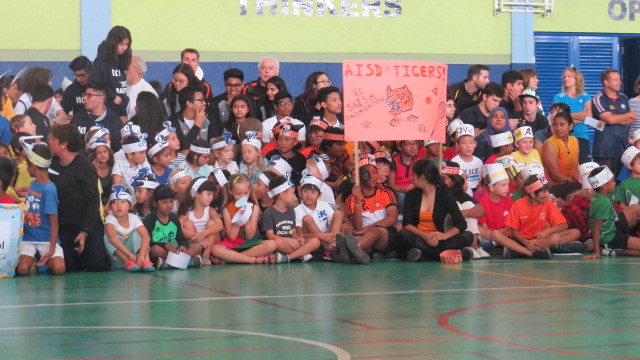The image depicts an event in a gymnasium, capturing a lively and colorful scene of a diverse group of children and a few adults. The gymnasium's green floor is crisscrossed with white, red, yellow, and blue lines, suggesting it is marked for various sports like basketball and volleyball. 

In the center of the image, two children are prominently holding a banner between them. The banner, with a pink background and red letters, reads "AISD Tigers," accompanied by a drawing of an orange tiger face, paw prints, and additional text such as "SAISA admission" flanking the sides. Surrounding these children are at least 100 more, sitting, standing, or kneeling on the floor, and some are on benches or chairs that rise towards the back, possibly forming a bleacher-like setup.

The children are wearing a rainbow of multicolored shirts, including green, white, gray, red, orange, and blue, along with white and blue paper headbands. The upper portion of the photo features a light green wall bordered by blue, with a blue double door to the right side. In front of this door stands a woman in a light blue jersey and a man in a gray and red jersey next to her. The letters "OP" in blue can be seen on the wall, adding to the school's decoration.

In the background, a group of adults stands behind the children, perhaps supervising or participating in what appears to be a school pep rally or an event celebrating the Tigers. The gymnasium walls are adorned with a mix of yellow, white-blue, and blue areas, adding to the festive atmosphere.